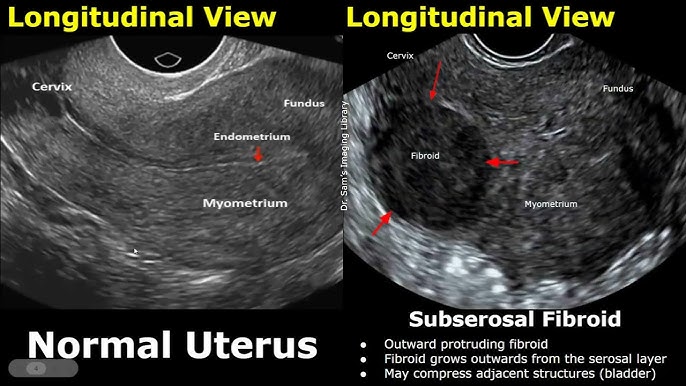The image displays two detailed ultrasounds of a woman's uterus, side by side, both marked with yellow text at the top indicating "longitudinal view." The left ultrasound, which is in black and white, is annotated with labels identifying the cervix, fundus, endometrium, and myometrium, with white text below stating "normal uterus." Conversely, the right ultrasound, also in black and white, identifies the cervix, fundus, myometrium, and specifically highlights a fibroid with three red arrows pointing to it. Below this ultrasound, white text indicates "subserosal fibroid," accompanied by bullet points that describe the fibroid as "outward protruding," "grows outward from the serosal layer," and "may compress adjacent structures like the bladder."